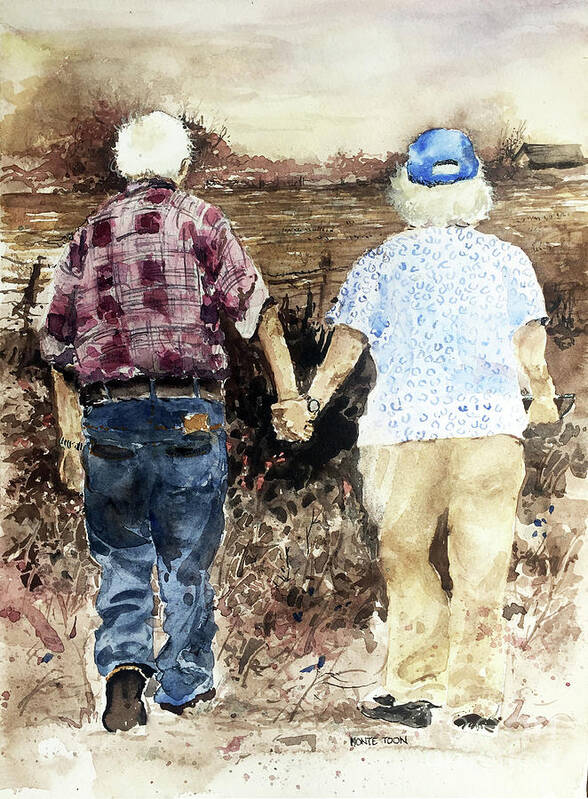This detailed painting portrays an elderly couple, viewed from behind, as they walk hand in hand, capturing a touching moment of companionship. On the left, the elderly man, with white hair, is dressed in a red plaid shirt with burgundy and darker red squares, dark blue jeans, brown shoes, and a watch on his left wrist. He also has a belt and a wallet visible in his back right pocket. His companion, the woman to his right, also has white hair and is wearing a cyan blue baseball cap. Her attire includes a cyan blue shirt adorned with U-shaped and circle-shaped outlines, beige pants, and black walking shoes. She, too, wears a watch on her left wrist. The couple stands before a bush, which displays shades of black and brown. They gaze upon their farm—a brown clearing dotted with trees and brush, including a tan farmhouse with a brown and gray roof to the upper right. The sky overhead is a blend of tan and gray hues. This tender scene is signed by the artist 'Monte Toon' at the bottom, beneath the woman’s feet.